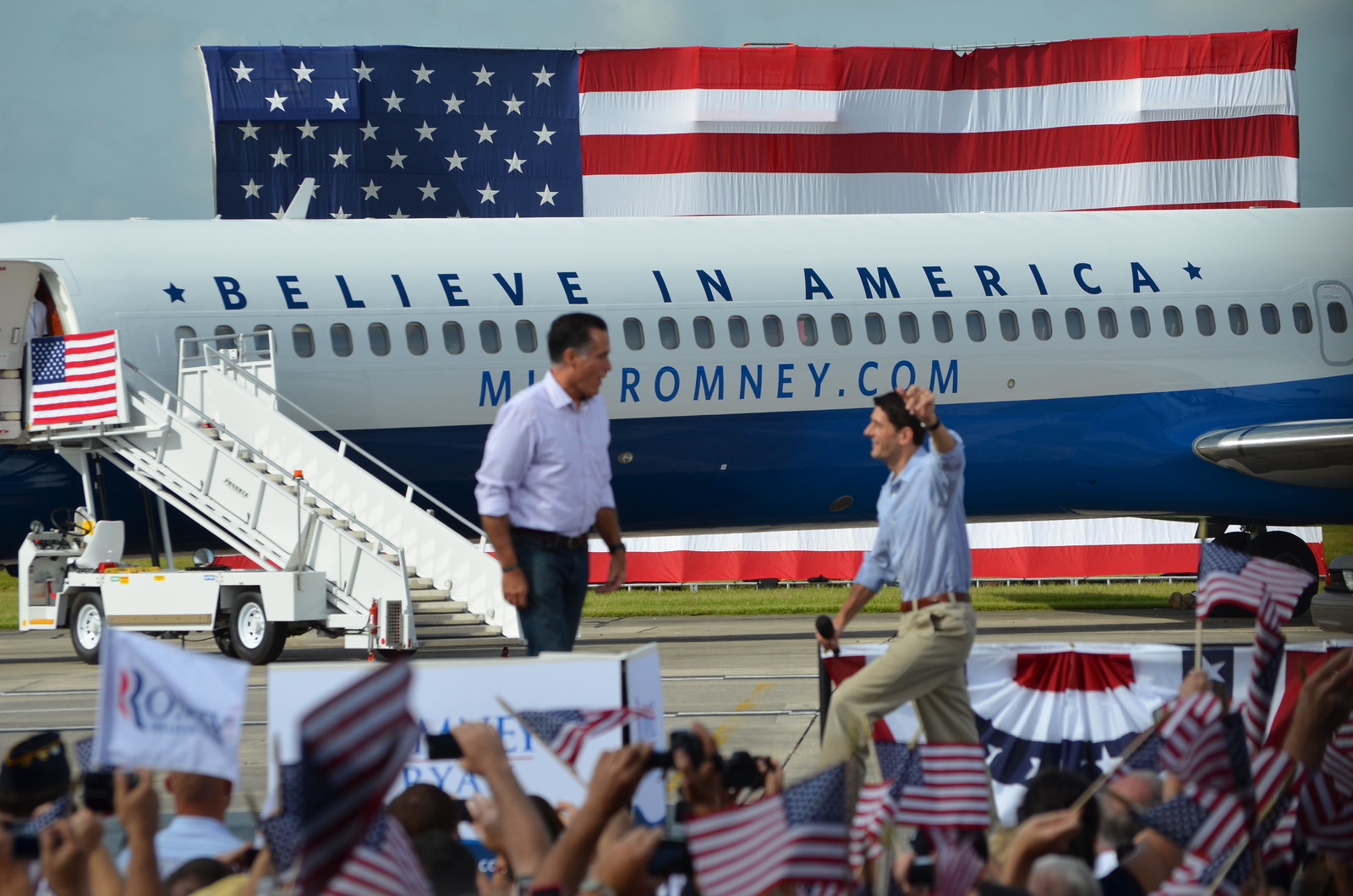This photograph captures a dynamic scene from a Republican political campaign event for Mitt Romney. In the foreground, Mitt Romney is seen walking towards a stage to greet another gentleman, both silhouetted against a backdrop featuring an aircraft. The aircraft prominently displays the slogan "Believe in America" along with the web address "MittRomney.com," though part of the word "Mitt" is obscured by Romney's presence. The top half of the plane is white and the bottom half is blue. Behind the aircraft and forming a dramatic backdrop is a large American flag, emblematic of the patriotic atmosphere. Surrounding the stage is a crowd of enthusiastic supporters, many waving American flags and holding up signs, some of which read "Romney" and possibly "Ryan." The event is taking place outdoors during the daytime, capturing the essence of a lively campaign rally.